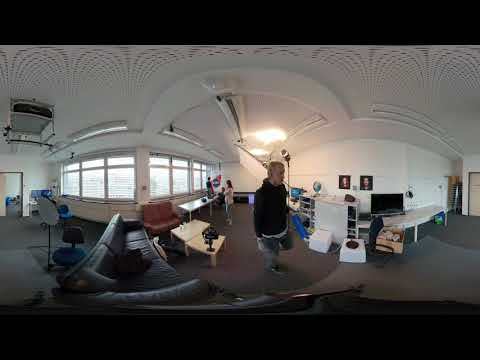The image depicts a panoramic view of a stark, plain office with white walls and a white ceiling, contrasted by gray carpeting throughout. The room is lined with seven windows, three on the left and four on the right, each adorned with horizontal blinds, some slightly parted to admit strips of light. The left foreground is dominated by a large, black couch facing right, beside which sits a small light-colored coffee table. Positioned above and to the right of the black couch is a smaller, reddish-brown loveseat. 

To the center of the image stands a man dressed in a black hoodie and gray pants, walking towards the right. His left leg is mid-step, knee jutting forward, while his right arm swings beside him. Near this figure, a woman gazes intently at a computer screen placed on a reflective silver table before her. Behind and to the right of the woman, a ceiling tile appears to be dislodged, hanging down precariously.

Further into the room, several white tables and storage units are grouped together, with some featuring solid fronts, possibly cabinets or shelves. A dark camera rests at the bottom right corner of the central coffee table. The scene extends to the far right, where a few portraits adorn the wall and a doorway is partially visible, suggesting another room beyond.